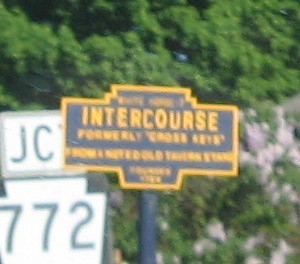This slightly blurry photograph captures a distinctive street sign set against a backdrop of lush, green, leafy trees. The primary sign is rectangular with ornate features, having a segment that slightly arches upwards in the middle at the top and dips down at the bottom. The sign is predominantly gray with yellow lettering and embellishments. At the very top, there is obscured text that is unreadable due to the blur. Below that, in large capital letters, the word "INTERCOURSE" stands out prominently. Directly beneath it, a subtitle reads "FORMERLY CROSS _____," though the last word is indiscernible. Further below, the sign contains additional lines of smaller text that are not readable. To the left of the main sign, there are two white street signs; one is partially obscured by the "INTERCOURSE" sign, showing only the letters "JC" and part of a "T." Below that, there is a small sign displaying the number "772" in gray lettering on a white background. The entire scene is framed by the verdant foliage of the surrounding trees.